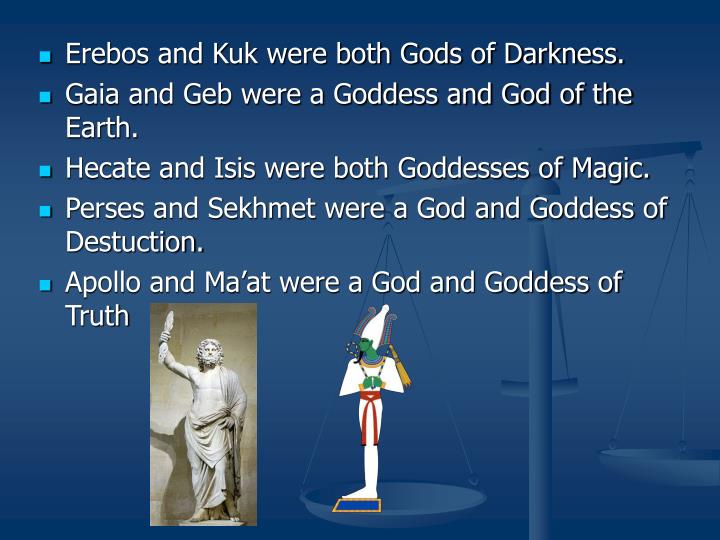The PowerPoint image features a blue background with text and images that compare different gods and goddesses. At the top, written in white letters on light blue bullet points, are five statements: 
1. "Erebos and Kuk were both gods of darkness."
2. "Gaia and Geb were a goddess and god of the earth."
3. "Hecate and Isis were both goddesses of magic."
4. "Perseus and Sekhmet were a god and goddess of destruction."
5. "Apollo and Maat were a god and goddess of truth."

Below these points, occupying the bottom middle section, are two images. On the left, a light grey statue of Zeus holding a lightning bolt, set against a blue background. The statue stands on a grey platform and is situated in a room with a tan wall. On the right, an illustrated depiction of the Egyptian god Osiris, who has a green face, green hands, and wears a white robe and cap, holding a flail and crook. Osiris is adorned with a red belt, a green and yellow necklace, and stands on a blue and yellow platform. Behind Osiris, to the far right, are blue scales of justice, balanced more heavily on the left side.